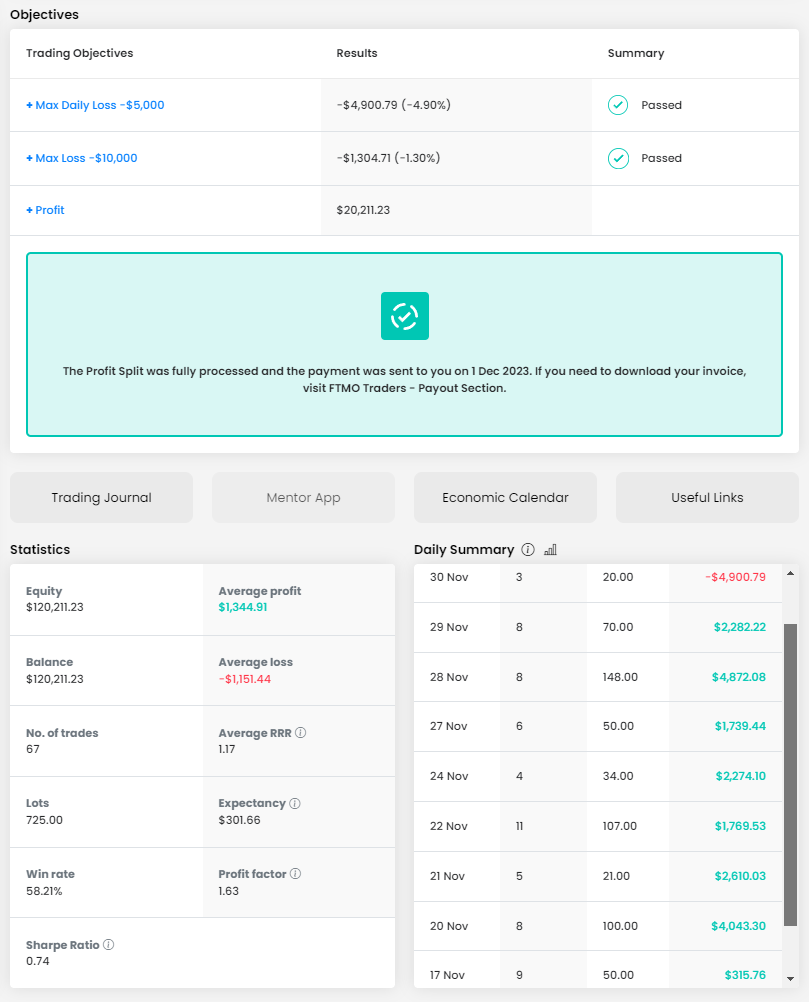This image showcases a digital application designed for tracking daily profits and trading activities, possibly related to stocks or similar investments. 

At the top left corner, the section titled "Objectives" is in bold black text. Directly beneath it is a box labeled "Trading Objectives, Results, and Summary," which contains a four-column, three-row table. Within this table:

- The "Trading Objectives" column lists:
  1. Max Daily Loss: -$5,000 (displayed in blue text)
  2. Max Loss: -$10,000 (displayed in blue text)
  3. Profit (displayed in blue text)

- The "Results" column provides the following data:
  1. -$4,979 (-4.90% in parentheses)
  2. -$1,304.71 (-1.30% in parentheses)
  3. $20,211.23

- The "Summary" column shows green check marks for both the Max Daily Loss and Max Loss objectives, indicating they have been passed. There is no summary entry for the Profit section.

Below this table, a green box with a green check mark states, "The profit split was fully processed, and the payment was sent to you on December 1st, 2023. If you need to download your invoice, visit the 'ftmotraders-payout' section."

Further down the interface, two adjacent boxes are displayed:
- The left box is titled "Statistics" and likely contains data such as equity and balance figures.
- The right box is labeled "Daily Summary," presumably detailing the profit for each individual day.

This detailed layout provides a comprehensive view of trading performance, objectives, and summaries, ensuring users can easily monitor and assess their financial activities.